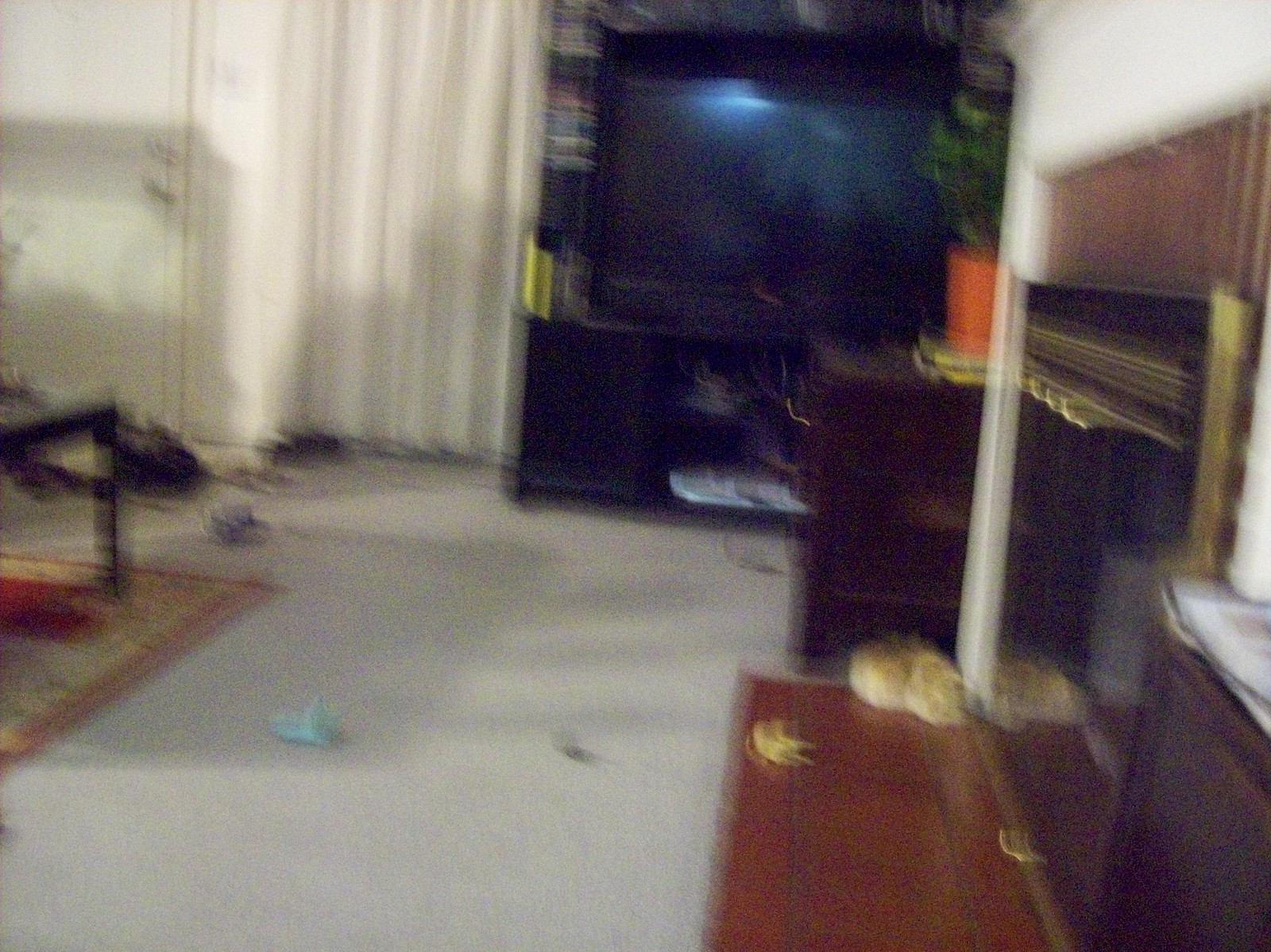The image depicts a very blurry and grainy photograph of a living room with multiple indistinct elements. Dominating the scene is a large television set placed within, or on top of, a black square entertainment center, situated at the end of a wall. Surrounding the TV are DVDs or CDs, though they're too blurry to identify clearly. To the right of the TV is a possible fireplace, which has a black cover and a brown hearth beneath a white mantel, and is possibly golden with brick detailing. In the background, some white curtains hang, possibly covering a door or window. Various indistinct objects are scattered across a grey or brownish rug on the floor. Additionally, there appears to be a brown end table or chest with a plant in an orange pot and other miscellaneous items, including something light blue, strewn about the room.